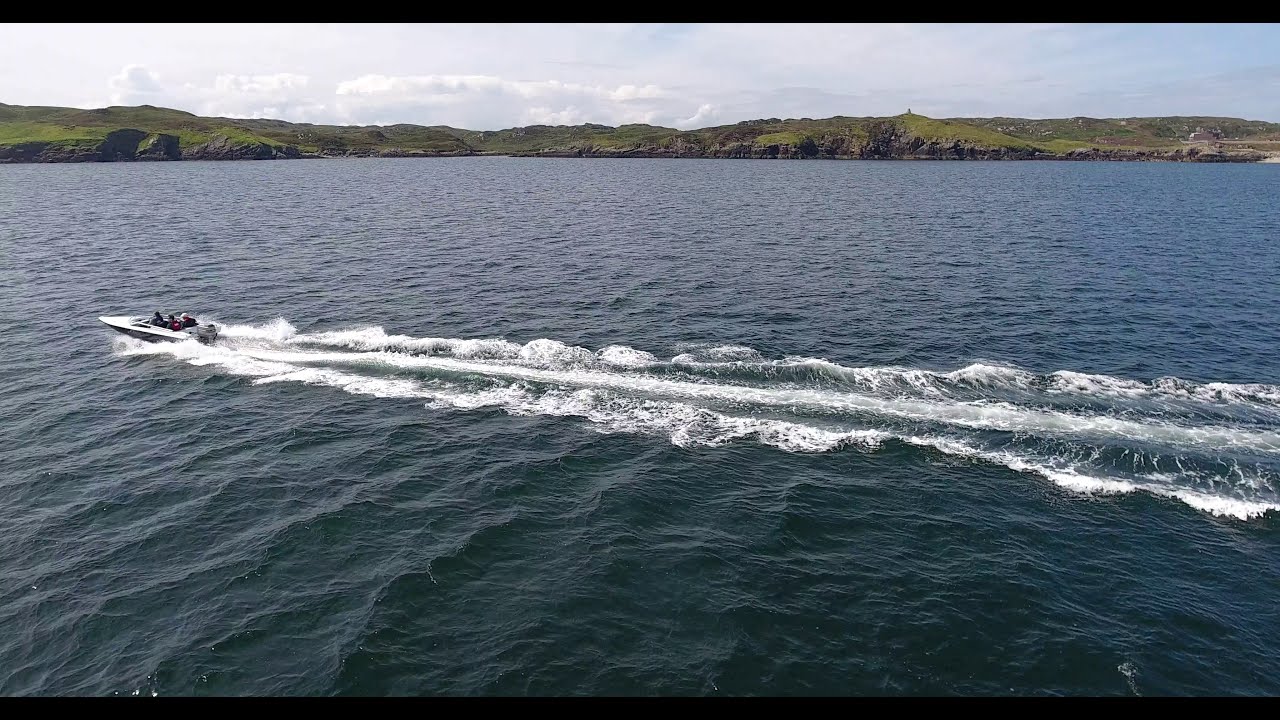A broad expanse of dark blue water sets the scene, with a speedboat prominently featured as it races from the right-hand side of the image toward the left. The boat, which is white and appears to be carrying three indistinct figures, kicks up a large, frothy wake that stretches across the water almost horizontally, leaving a wide, white streak that disrupts the otherwise calm surface. The sky above is a white-gray shade, filled with clouds, while the distant horizon reveals green, grassy hills capped with shrubs and dotted with traces of buildings. Rocky cliffs with gray and brown hues form a rugged shoreline, adding to the landscape's contrast and depth.